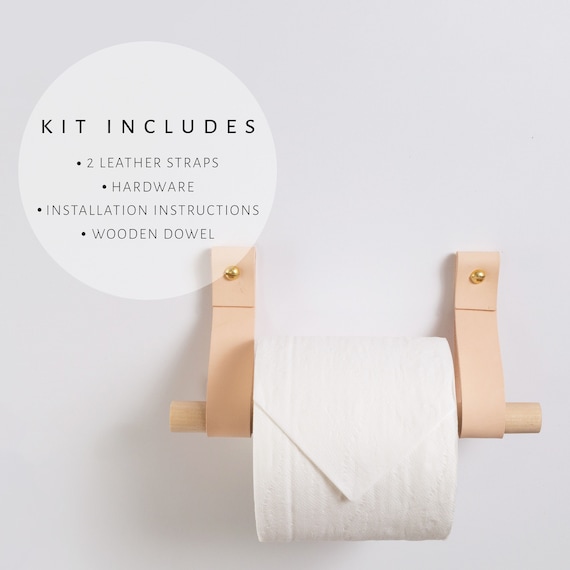This image is an advertisement for a minimalist toilet paper roll dispenser kit designed for home use. The dispenser is displayed against a plain gray background, showcasing two light tan, almost beige, leather straps mounted on the wall with small brass fasteners. These straps hold a wooden dowel, which in turn suspends a roll of toilet paper. The text to the left of the image is enclosed within a circle and details the kit’s contents in capital letters, each item separated by a dot and listed on separate lines. The kit includes two leather straps, hardware, installation instructions, and a wooden dowel. The toilet paper roll on the dowel is intricately pointed at the end, demonstrating practical usage and adding to the overall aesthetic of the design.